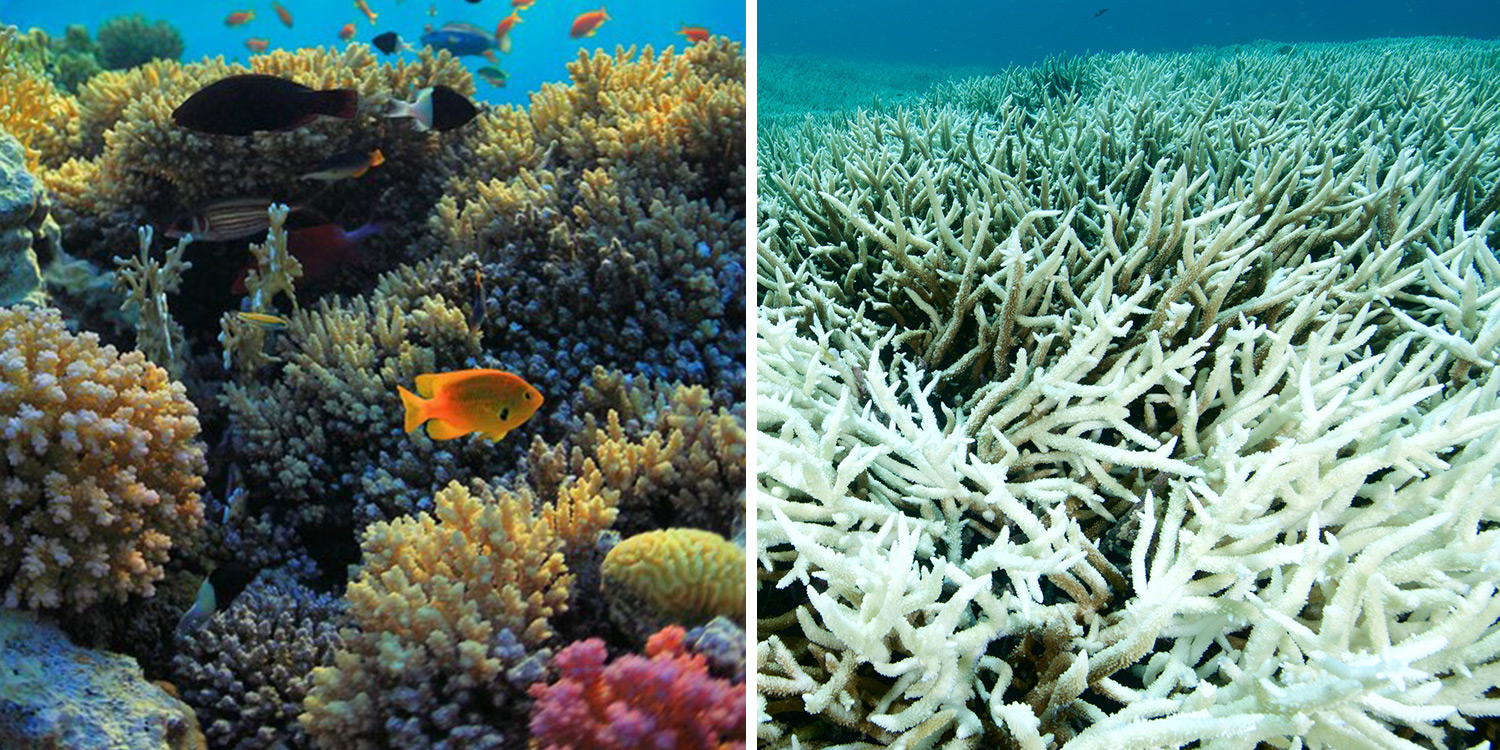The collage comprises two side-by-side underwater scenes displaying contrasting marine environments. The left photograph bursts with colorful corals, showcasing shades of yellow, blue, pink, and red. Among the corals, a variety of fish swim gracefully. A bright orange fish is nearest to the camera, accompanied by a very dark, possibly black or dark red fish, and a half black, half white fish. Further afield, more orange and blue fish are visible, contributing to the teeming aquatic life. In this vibrant setting, different corals, rocks, and diverse life forms create a lively underwater landscape. In stark contrast, the right photograph features an expansive view of bleached coral, predominantly white and stretching far into the background. This depiction of bleached coral highlights environmental concerns such as global warming, which is significantly impacting oceanic ecosystems. The further the corals recede, the greener their tones become, eventually blending into the darker blue hue of the distant ocean.